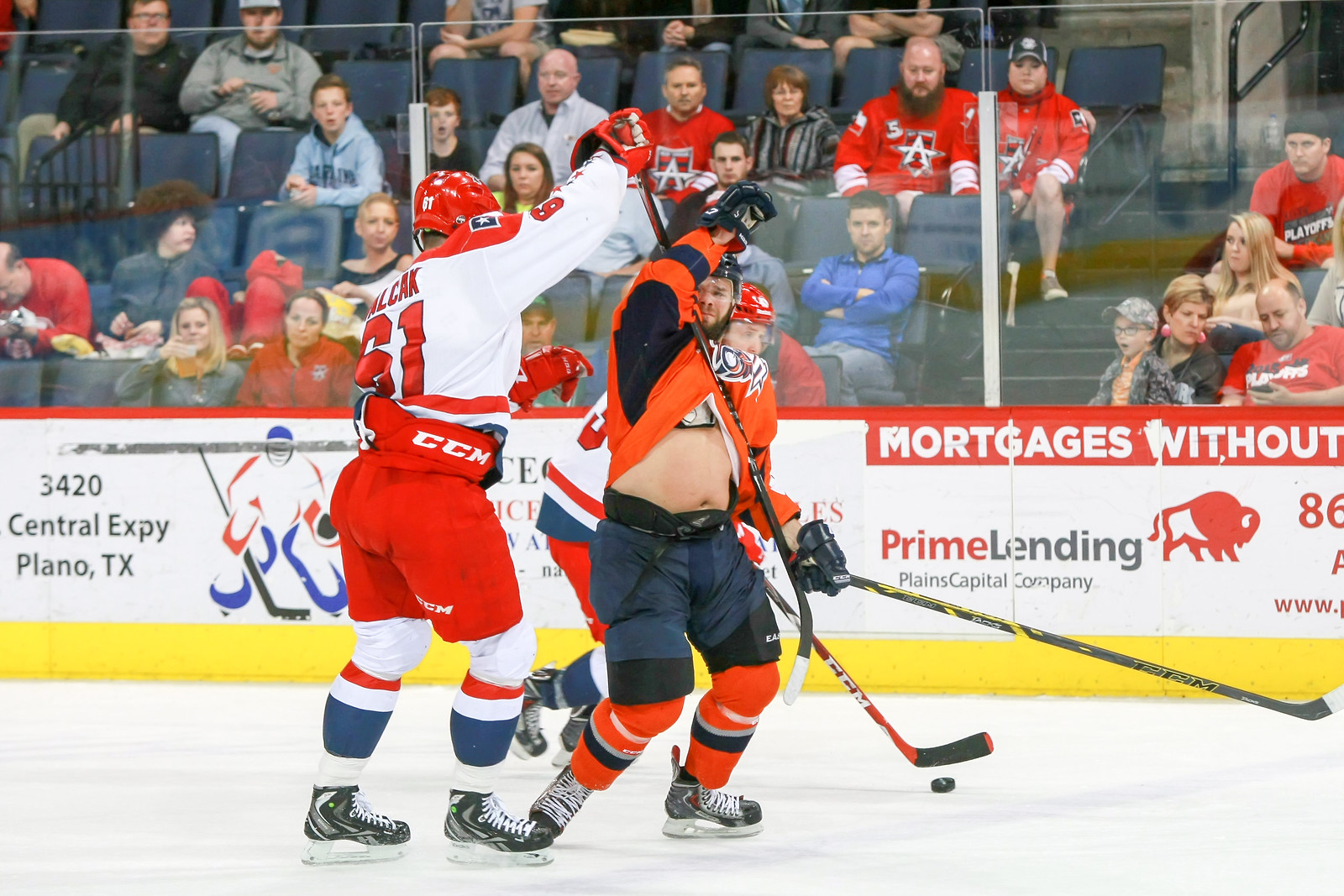In this action-packed hockey scene, two prominent players are in focus on the ice, surrounded by an animated crowd. The player on the left, distinguishable by his predominantly white and red uniform with blue, white, and red-striped socks, has his hockey stick raised in the air. His red shorts and red details on his jersey emphasize his team's colors. To his right, an opposing player wears an orange and white uniform, including blue pants and orange knee pads, and appears to be hooking his arm around the white and red player's raised stick, looking concerned. Behind them, a third player from the white-and-red team skates towards the action while controlling the puck. The background features two partially obscured advertisements, one for "Prime Lending, Plains Capital Company" promoting "Mortgages Without," and another indicating "3420 Central Expressway, Plano, Texas." The crowd, largely outfitted in red jerseys, suggests strong support for the home team.